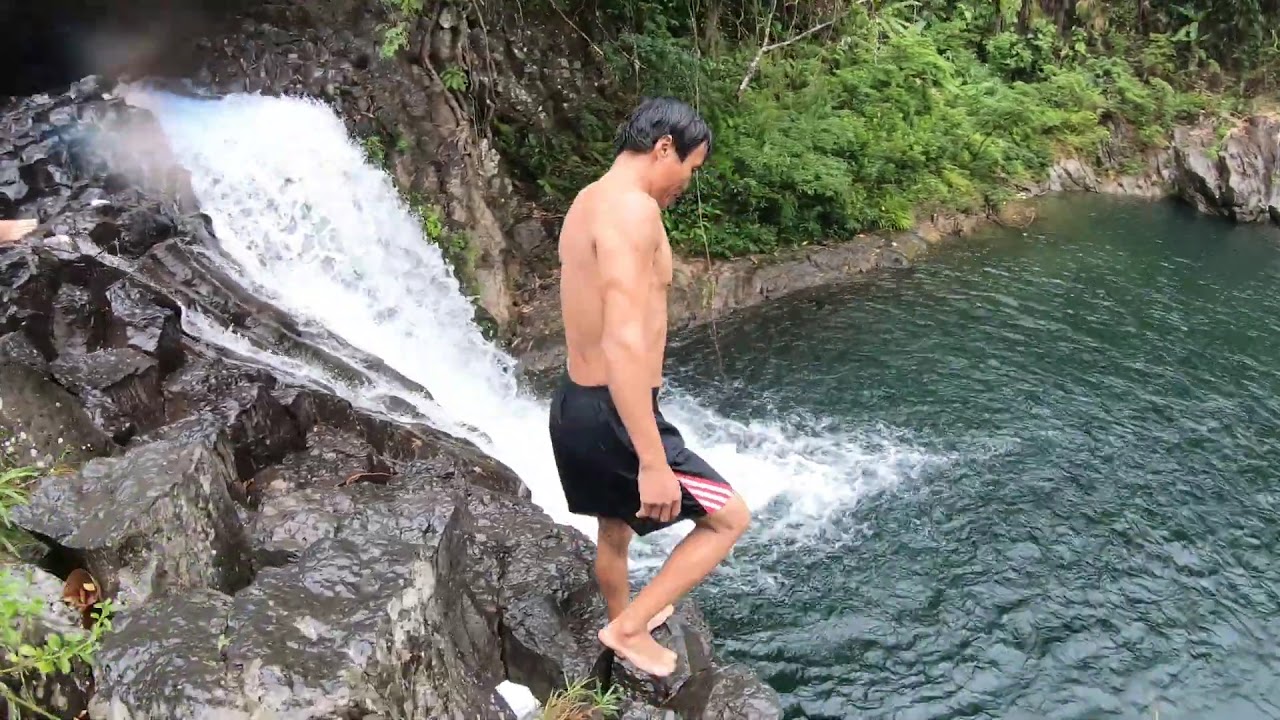A young man with dark hair stands on a rocky slope of a bluff, poised to jump into a vibrant teal pond below. He is wearing black swimming trunks with white and red accents and is looking down intently. Beside him, a small waterfall cascades into the pond, creating a striking white contrast against the darker colors of the water. Surrounding the scene, vivid green shrubbery and trees dot the shore, adding lushness to the landscape. The light quality suggests a hazy or semi-overcast day, but the colors of the image remain exceptionally bright and clear, enhancing the overall vividness of this picturesque moment.